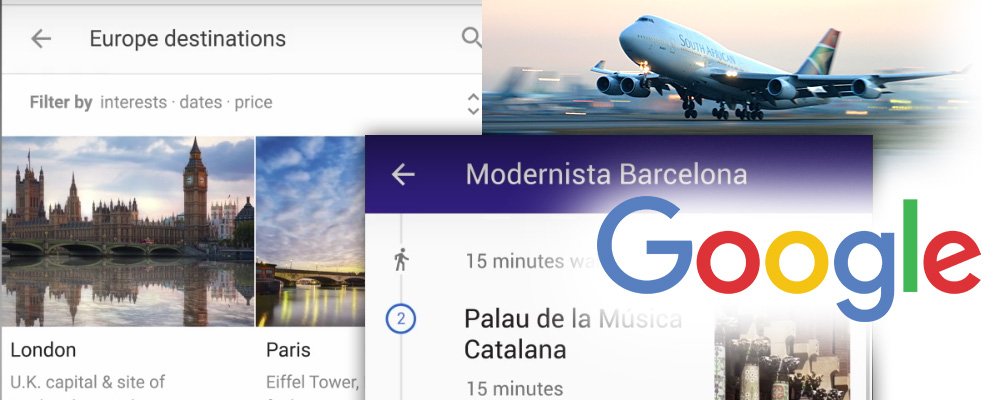The image depicts a composite web page with various overlapping elements, creating a chaotic, collage-like appearance. In the upper left-hand corner, there is a back button next to the heading "Europe destinations." To the right of this heading, there are icons including a search symbol and an image of a plane taking off, specifically a South African Airways plane. Below them, there are filtering options labeled "Filter by interests, dates, and price." 

In the main body of the page, several destination images are displayed. One shows London with a picture of what appears to be St. Paul's Cathedral, captioned "London: UK Capital." Another picture showcases Paris with a focus on one of its iconic bridges. However, much of this image is obscured by an overlapping window.

This overlapping window contains another back button and a purple bar with white lettering reading "Modernista Barcelona." It seems to provide walking directions, stating a "15-minute walk," but much of this information is covered by a prominent Google logo positioned in the bottom right corner. The text "Palau de la Música Catalana, 15 minutes" is also partially visible under the Google logo.

Overall, the image resembles a haphazardly assembled digital collage, reminiscent of a poorly constructed scrapbook page filled with various, uncoordinated web elements.